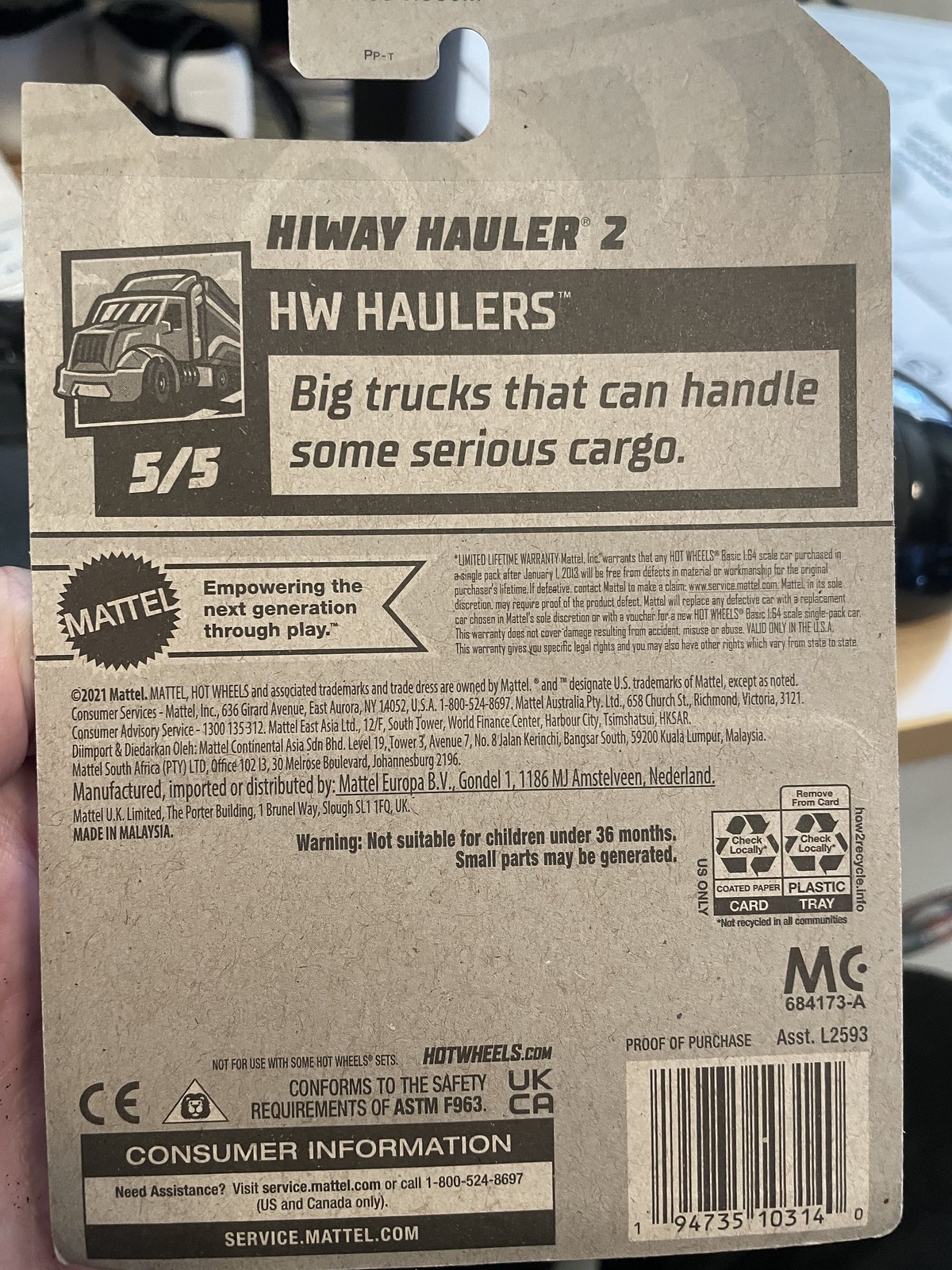The image shows the back of a toy package, likely from Mattel's Hot Wheels or Matchbox series. Dominating the cardboard backing is the prominent text "Highway Hauler 2" at the top. Below this title, there's a sketch of a semi-truck, partially visible. The black banner reading "HW Haulers" stands out, followed by the slogan "Big trucks that can handle some serious cargo." To the left is a black area displaying "5/5" in white print. Beneath this, you can find the iconic Mattel logo in a circle with sun-like edges, accompanied by their slogan "empowering the next generation through play."

Additional small print around the package includes consumer information, a warning about suitability for children under 36 months due to small parts, and a UPC code in the bottom right corner. The text also details a limited lifetime warranty for Hot Wheels Basic 1:64 scale models purchased after January 1, 2013, emphasizing coverage for material or workmanship defects and instructions for making a warranty claim.